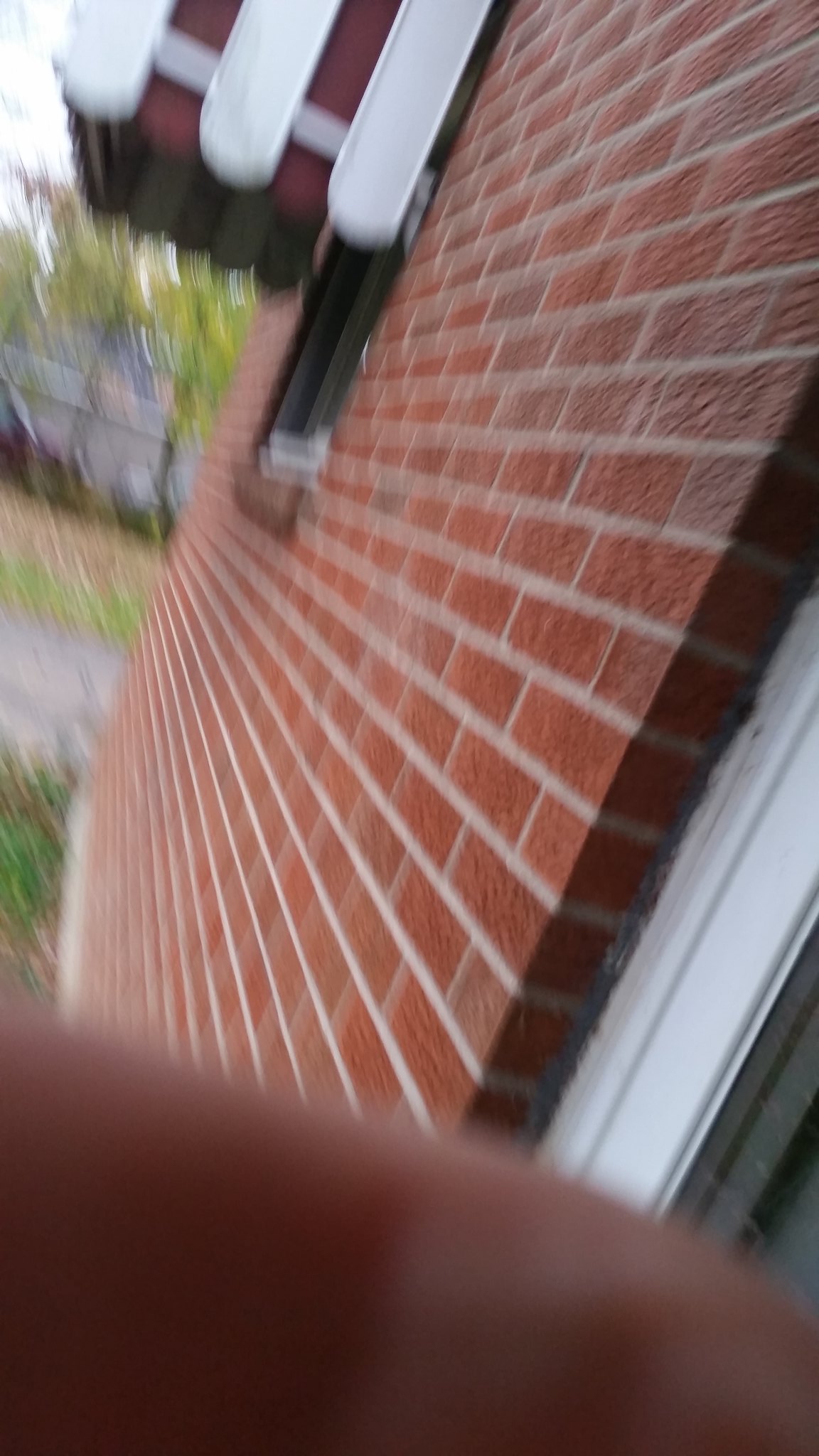In the background, a serene forest of verdant trees provides a lush backdrop. Beneath the foliage, a stone wall stretches across the scene, bordered by a leaf-strewn ground and a weathered stone sidewalk. Prominently featured is a quaint, rustic wall constructed from numerous bricks, each delineated by white mortar lines that create a pattern of division. Adjacent to the bricks, sections of white wood frame a window, adorned at the top with what appears to be a decorative array of white, popsicle stick-like elements. In the foreground, a finger partially obscures the lens, adding an inadvertent, human touch to the composition.